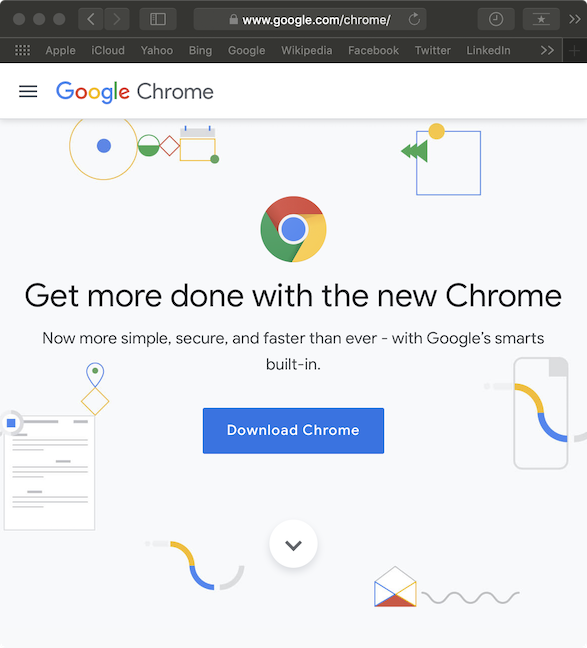The image is a screenshot of a web page viewed in Google Chrome. At the top of the page, there is a black banner featuring several tabs labeled with various website names: Apple Cloud, Yahoo, Bing, Google, Wikipedia, Facebook, Twitter, and LinkedIn. Below this banner, "Google Chrome" is prominently displayed.

The Google Chrome browser icon is visible, shaped like a circular donut with colors transitioning in a sequence of green, yellow, and red, surrounding a blue circle in the center. Next to the Chrome icon, text reads, "Get more done with the new Chrome: simpler, more secure, and faster than ever with Google smarts built-in." At the bottom of the page, a button prompts users with the call to action, "Download Chrome."